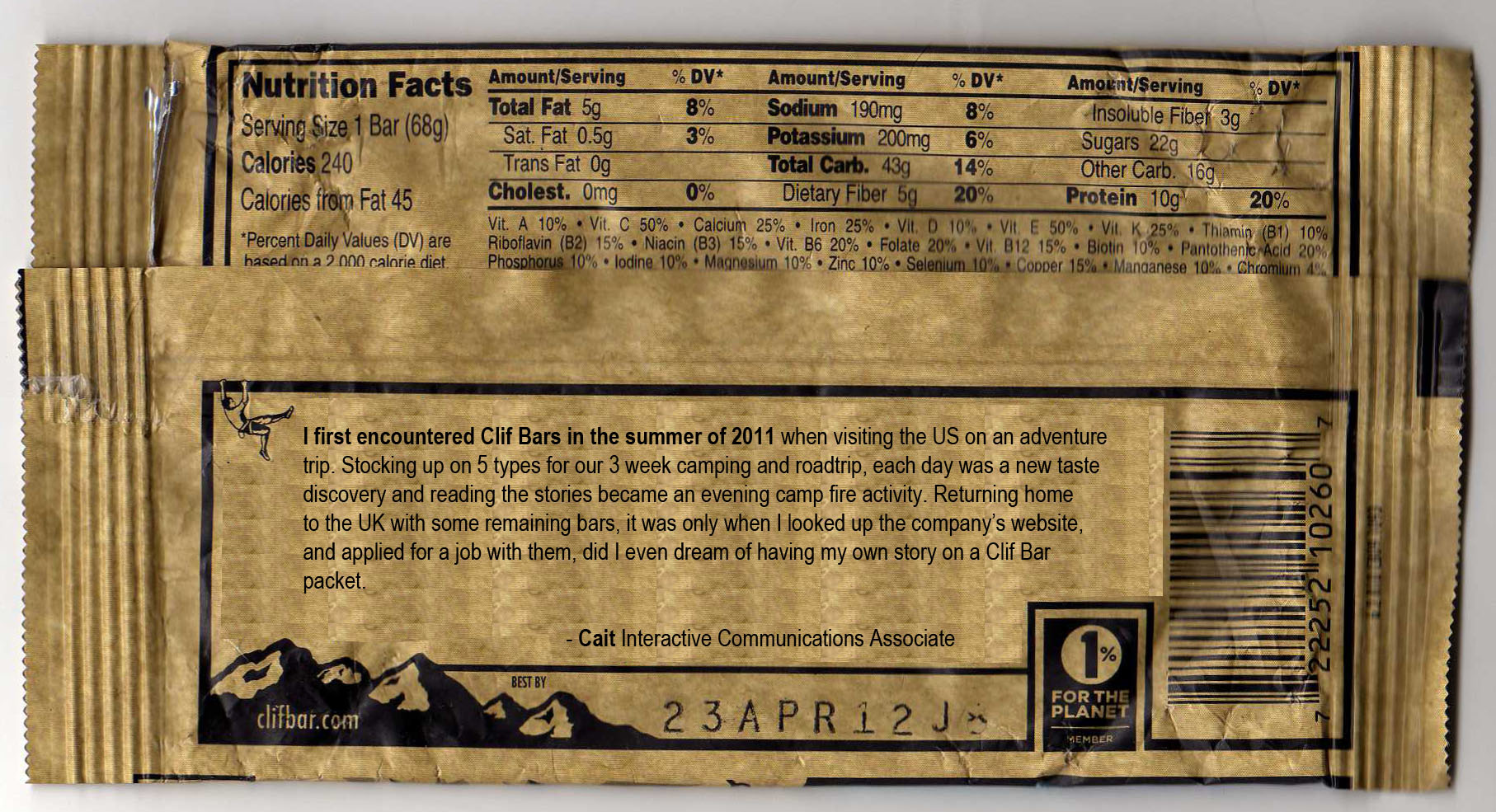The image showcases the back of a gold-colored Clif Bar wrapper, featuring comprehensive nutritional information. The nutrition facts panel details the serving size, calorie count, and the amounts of total fat, cholesterol, sodium, potassium, total carbohydrates, and protein. Additionally, a significant date, April 23, 2012, is printed on the wrapper, possibly indicating the production or expiration date. Alongside this information, the wrapper lists a website, clifbar.com, for further product details. The nutritional facts and some product information are displayed within a black rectangle, contrasting against the gold background. There is also a mention of an individual's first encounter with Clif Bars dating back to the summer of 2011, adding a personal touch to the otherwise informative packaging.